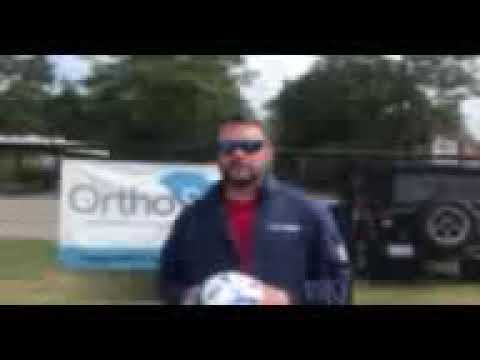The image is a blurry, grainy daytime photograph with black horizontal bars at the top and bottom, creating distinct black stripes. In the center of the photo, a man of Caucasian descent stands facing the camera from about the waist up. He has very short brown hair, a mustache, and a beard with possible gray streaks. He wears dark sunglasses, a red t-shirt, and a partially open black or dark blue long-sleeved jacket. He holds a white, round object in his slightly raised hands, but the image quality makes the object indistinguishable. 

To the man's right in the background, there is a black Jeep Wrangler with a rear spare tire visible. On his left side, a white banner with blue accents and "Ortho" written in black font hangs, possibly on a fence. Behind him is a clear blue sky with trees reaching into the frame.